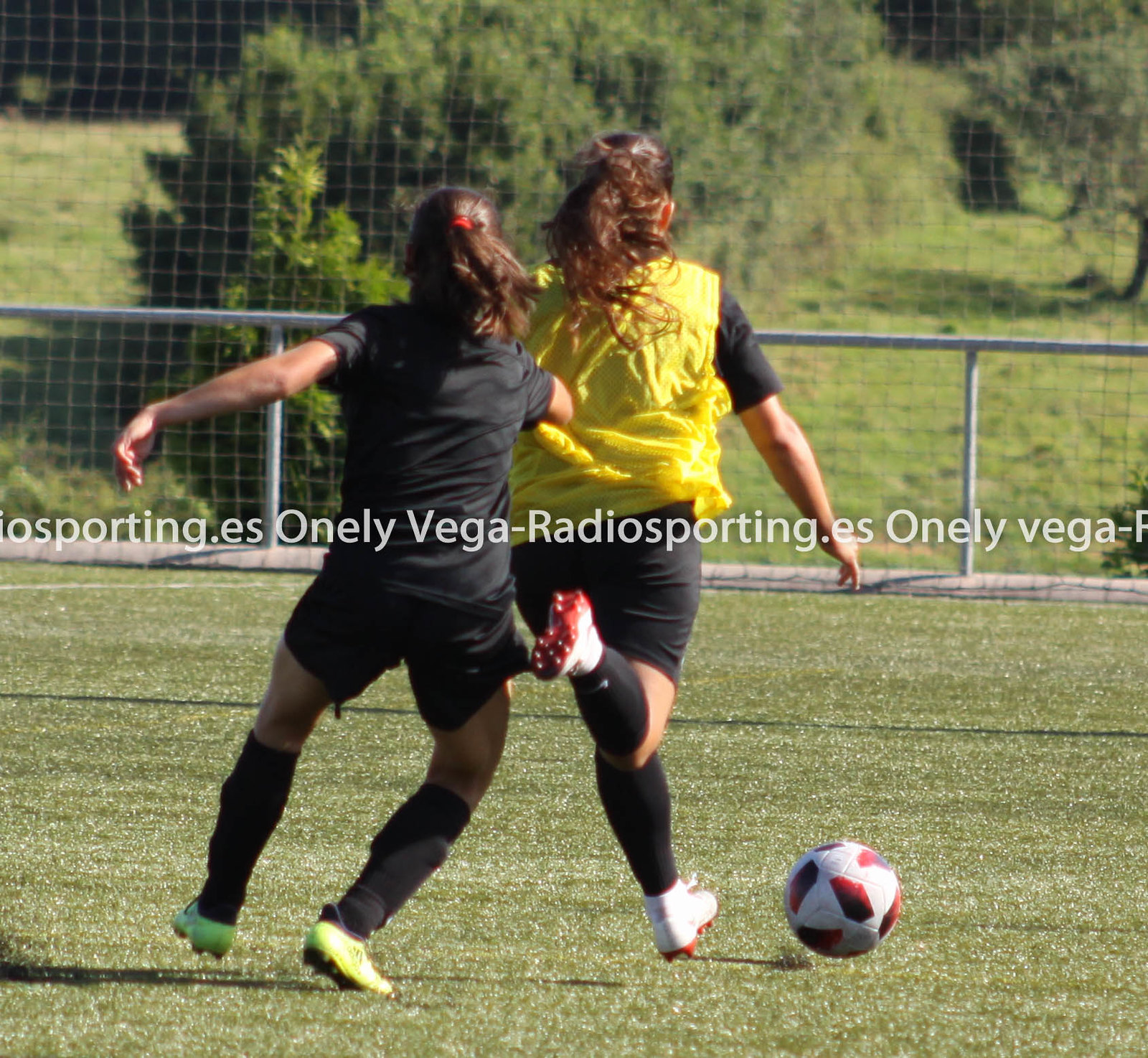The image depicts the intense moment of two women engaged in a soccer match, captured from behind. The focus is on their efforts to control a white soccer ball adorned with red patterns, positioned to the right of them on a shiny turf field, under an outdoor setting. Both women sport long hair tied in low ponytails and are in strikingly similar athletic gear—black jerseys, black shorts, and black socks. The woman on the left, distinguished by her yellow vest over her black outfit, is reaching out in an attempt to catch up to her opponent. Conversely, the woman on the right, also wearing a yellow vest over her black jersey and black socks but with white shorts, is in close pursuit of the ball. Surrounding them is a metal fence with netting designed to keep the ball in play, beyond which lie hilly terrain adorned with shrubs and trees. The scene is overlayed with text, twice reading "OneLeagueVega - RadioSporting.es," and partially visible lettering that seems to spell out “Vigor Radiosporting.es.”